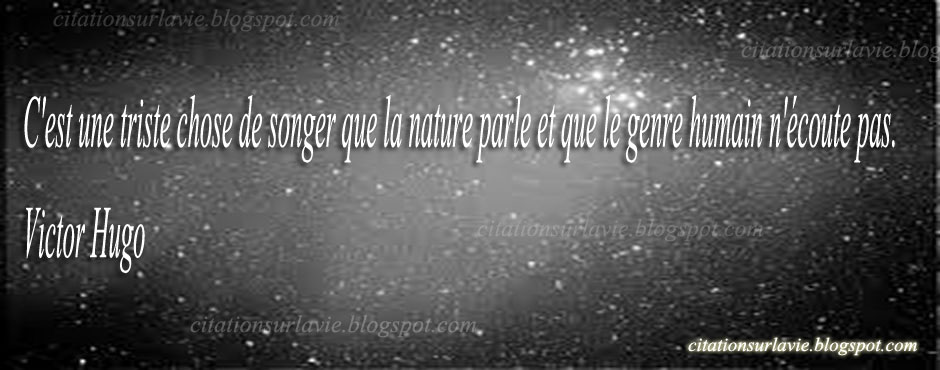This image features a quote by Victor Hugo set against a gradient background that emanates from the center. The gradient starts with a light gray in the very center, transitions to a darker gray, and finally to a black border. Scattered throughout the background are numerous white dots, giving it a space-like, celestial appearance. In the bottom right corner, "Citation SirLevy.blogspot.com" is subtly written in a very faint yellow color and small font. 

About a third of the way down the image, a row of white text in a serif font presents the quote in French: "C'est une triste chose de songer que la nature parle et que le genre humain n'écoute pas," which translates to "It is a sad thing to think that nature speaks and that humankind does not listen." Directly beneath the quote is the attribution "Victor Hugo," also in the same white serif font. The text stands out against the dark and starry background, adding a poignant touch to the visual.